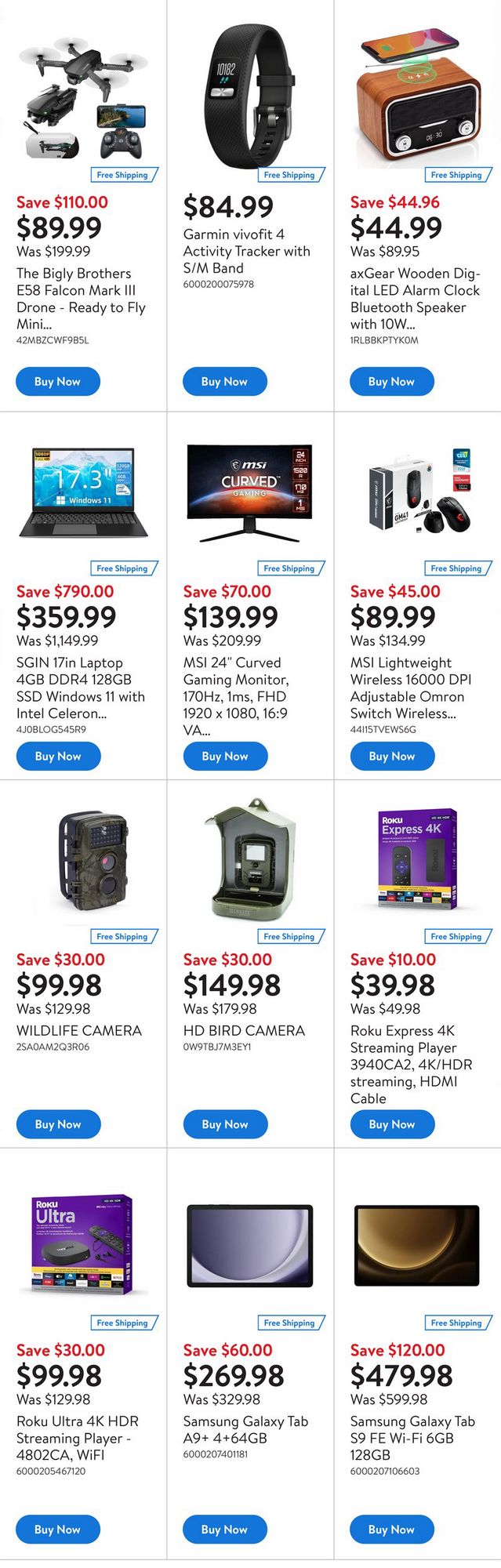The image displays an online marketplace with products for sale. The layout consists of four rows and three columns of items. Here are the details for the first two rows:

#### Top Row:
1. **Bigley Brothers E558 Falcon Mark III Drone**:
   - **Discount**: Save $110
   - **New Price**: $89.99 (Original Price: $199.99)
   - **Description**: Ready to fly, mini drone
   - **Additional Info**: Free shipping
   - **Action**: "Buy Now" button in blue
   - **Image**: Photo of the drone

2. **Garmin VioFit 4 Activity Tracker**:
   - **Price**: $84.99
   - **Spec**: Comes with S/M band
   - **Action**: "Buy Now" button
   - **Additional Info**: Free shipping
   - **Image**: Photo of the activity tracker

3. **AX Gear Wooden Digital LED Alarm Clock**:
   - **Discount**: Save $44.96
   - **New Price**: $44.99 (Original Price: $89.95)
   - **Spec**: Alarm clock with Bluetooth speaker, 10W
   - **Action**: "Buy Now" button
   - **Image**: Image of the alarm clock

#### Second Row:
1. **Sgin 17-inch Laptop**:
   - **Discount**: Save $790
   - **New Price**: $359.99 (Original Price: $1,149.99)
   - **Spec**: 4GB DDR4 RAM
   - **Additional Info**: No further details detected

Each item has a clearly marked price, discount, and a "Buy Now" button, with supplementary images and details to engage potential buyers.